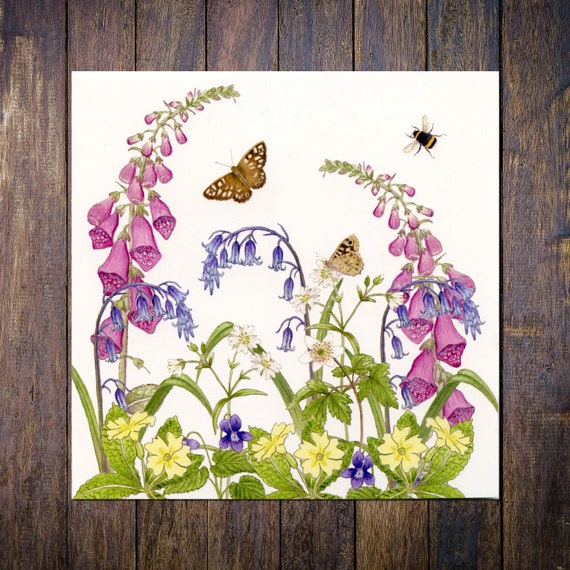A square watercolor painting is set against dark, vertically laid wooden floorboards, possibly made of oak. The white square canvas features a detailed and vibrant array of flora and fauna. At the forefront are yellow primroses, delicate and pale, nestled among assorted purple flowers, including both light and dark violet shades. Towering over these are majestic foxgloves with light green stems and pinkish-lilac buds. Alongside them are bluebells, their long stems adorned with individual, drooping blue flowers.

The natural scene is animated with wildlife; a bumblebee hovers in the upper right corner, while two butterflies add dynamic interest. One butterfly, in flight, is gold with white, hole-like patterns on its wings, and another rests on a flower, beige with black markings. The flowers are complemented by occasional sporadic bluebells and rich green leaves, adding to the vivid color palette that ranges from pinks and purples to yellows and greens. The butterflies may appear brown and understated, yet they contribute to the natural beauty of the composition. Overall, the painting evokes a serene and lively garden scene, capturing the vibrant essence of nature in watercolor.